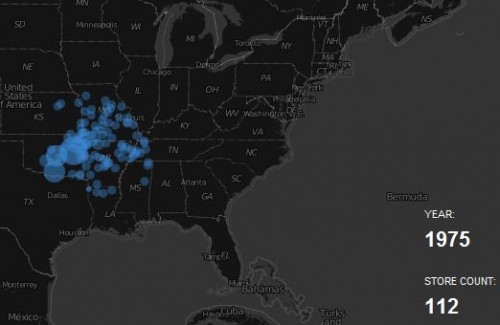In this rectangular illustration, we see a stylized map of the United States and portions of North America. The map is set against a gray backdrop where the lower half depicts water. The map's borders are outlined in black and light gray, emphasizing the United States while also including parts of Mexico and Canada. Notably, there are numerous blue blurry dots concentrated in the Midwest, which appear to represent some form of data, likely store locations. In the lower right corner, above the expanse of water, prominent white text reads, "Year 1975," and below it, "Store count: 112." While the blue dots are highly blurred, they seem to indicate a significant presence of stores, particularly clustered in the Midwest region.